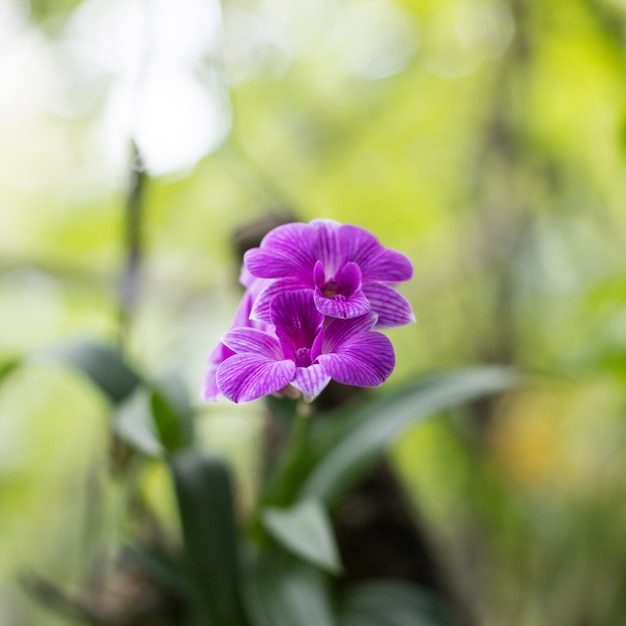This photograph captures an intimate close-up of two blooming purple flowers, possibly in a garden setting. The focal point of the image is on these flowers, which display a rich purple hue accented by white stripes along the petals. Each flower features approximately six larger petals, with smaller inner petals forming a delicate bud-like center. Hints of yellow, perhaps nectar, are visible within the blossoms. The flowers appear to share a green stem, with slender, spear-shaped leaves that elongate to pointy tips. The background fades into a blur, casting abstract patches of dark and light green with some white, contributing to the overall impression that it might be summer or spring. Bright spots, potentially sunlight or other flora, add an ethereal touch to the upper left corner of the image.